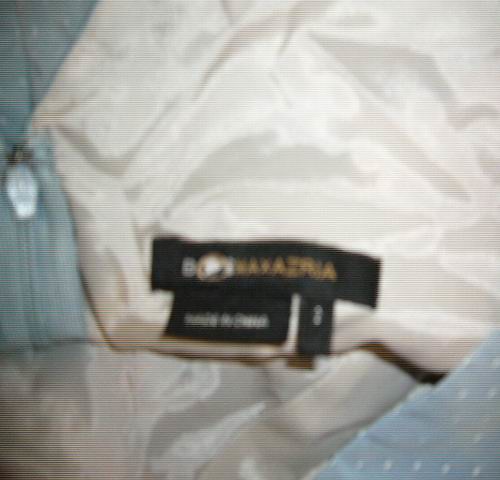This image, with its square orientation, exhibits notably poor quality characterized by low resolution and pixelation. Central to the composition, there is a black label displaying text in white and yellow hues. Beneath this primary label, two additional labels are discernible, despite the blurriness. The label on the left features white text but is not clearly legible, while the thinner label on the right also hosts white text. The background appears predominantly white, with an indistinct object on the left side further contributing to the lack of clarity in the image.